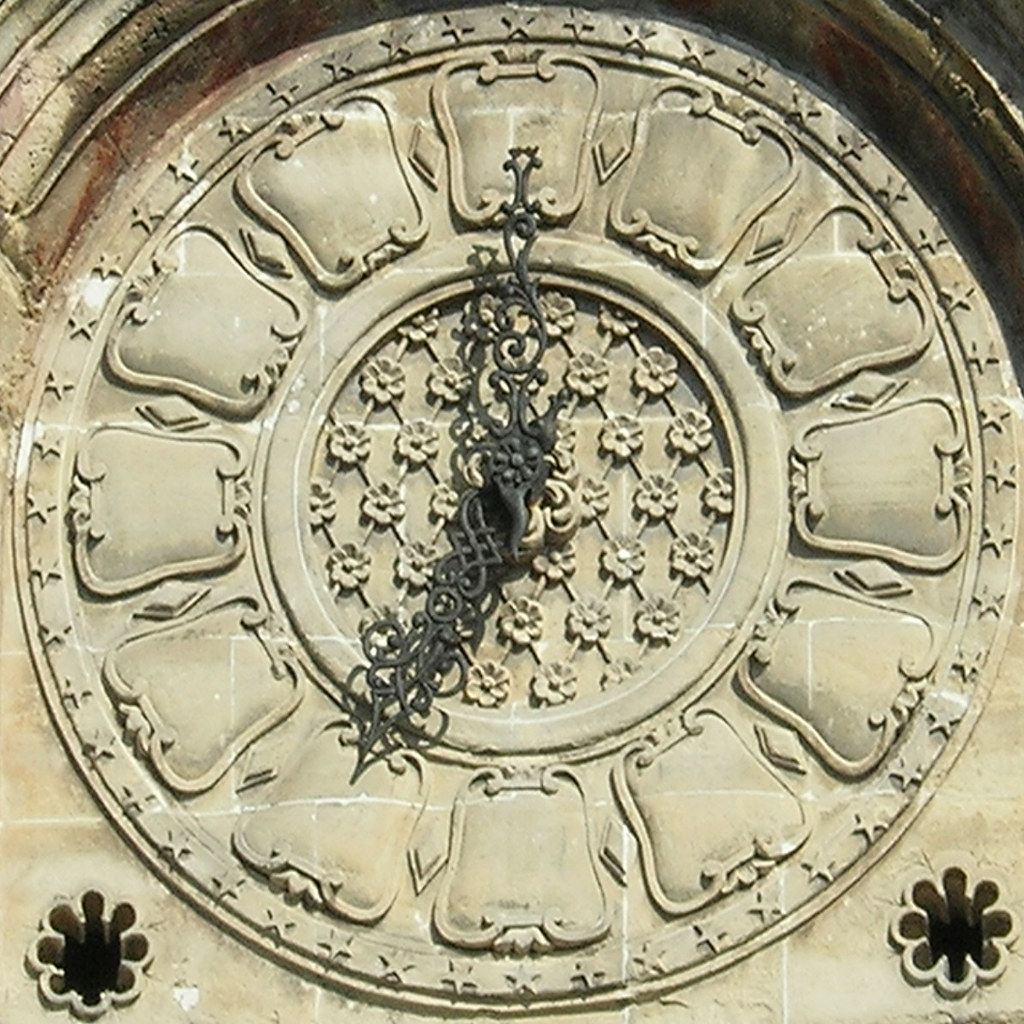This image showcases a distinctive clock face that is seamlessly integrated into a stone building. The clock dial, made entirely of a gray stone material resembling cement, features a unique and intricate design. At the center of the clock, the black hands—crafted with an ornate, thorny appearance—indicate the time, though no second hand is present. Encompassing the clock hands, a circular, flower-like pattern adds an artistic touch to the dial's center. Instead of traditional numbers, the clock uses square markers, each modified with a frame-like design at the top and bottom, maintaining the uniform gray stone color. Additionally, the clock's border is adorned with small star-shaped decorations, enhancing its overall aesthetic and blending harmoniously with the architectural style of the building.